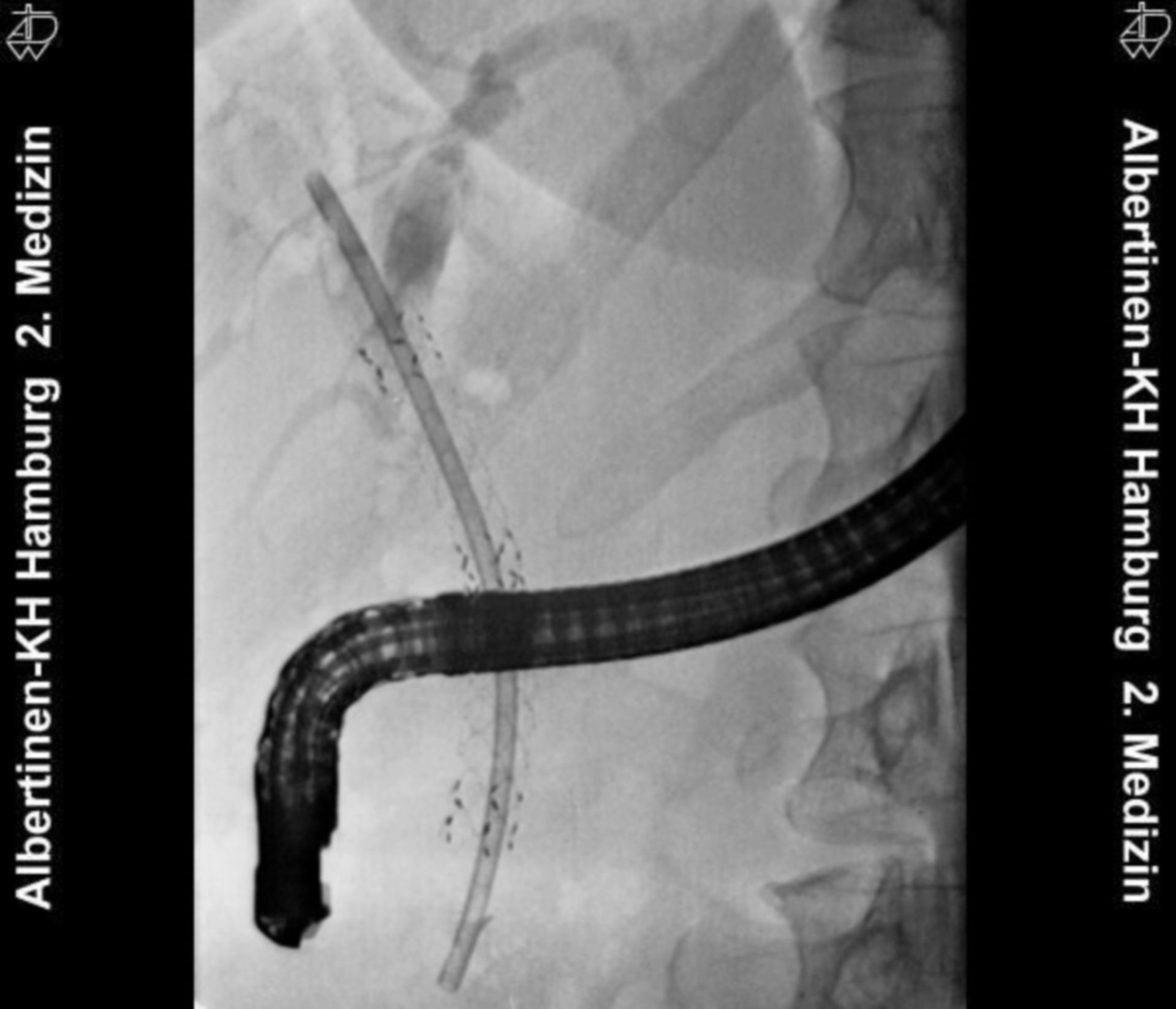This black-and-white image, oriented sideways, appears to be an X-ray. On both the left and right sides, there are solid black strips with vertically aligned white text reading "Albertinen K.H. Hamburg II Medicine." The main subject of the image, against a horizontally aligned, crinkled white background, is a dark, tube-like object resembling a snake or a worm. This object emerges from the right side, curving centrally and downward towards the lower left. The object has coil-like sections or segments, and there are additional thin, gray strands visible behind it. The overall setting suggests a medical context, possibly depicting an internal body part or a medical instrument within an X-ray scan.